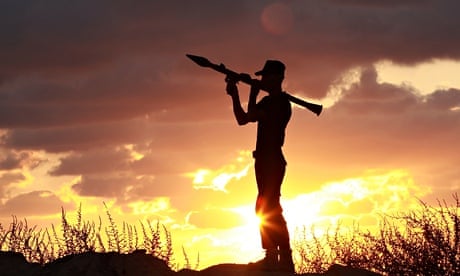In this richly detailed silhouette photo, the main focus is a lone figure, likely a marine or soldier, standing prominently against a dramatic sky at either dusk or dawn. The man, positioned in the center of the small rectangular image, is holding a rocket launcher on his shoulder, with his right hand on the barrel and his left hand on the trigger. He is facing to the left, his back slightly turned to the right. The soldier's form is rendered as a dark silhouette, making it impossible to discern any facial features, but one can clearly see that he is wearing a hat with a brim, pants, and boots.

The composition also includes elements of the natural world. The ground beneath him appears rocky, with sparse patches of grass and weeds visible at the bottom corners of the image. The sky forms a stunning backdrop, with clouds in shades of dark red to gray giving way to bright sunlight near the horizon, hinting at the setting or rising sun. The sky's color gradient shifts from a pinkish hue at the top to a yellowish glow closer to the rocky terrain, adding depth and atmosphere to the scene. This image captures a moment of solitude and readiness, framed by the raw beauty of nature.